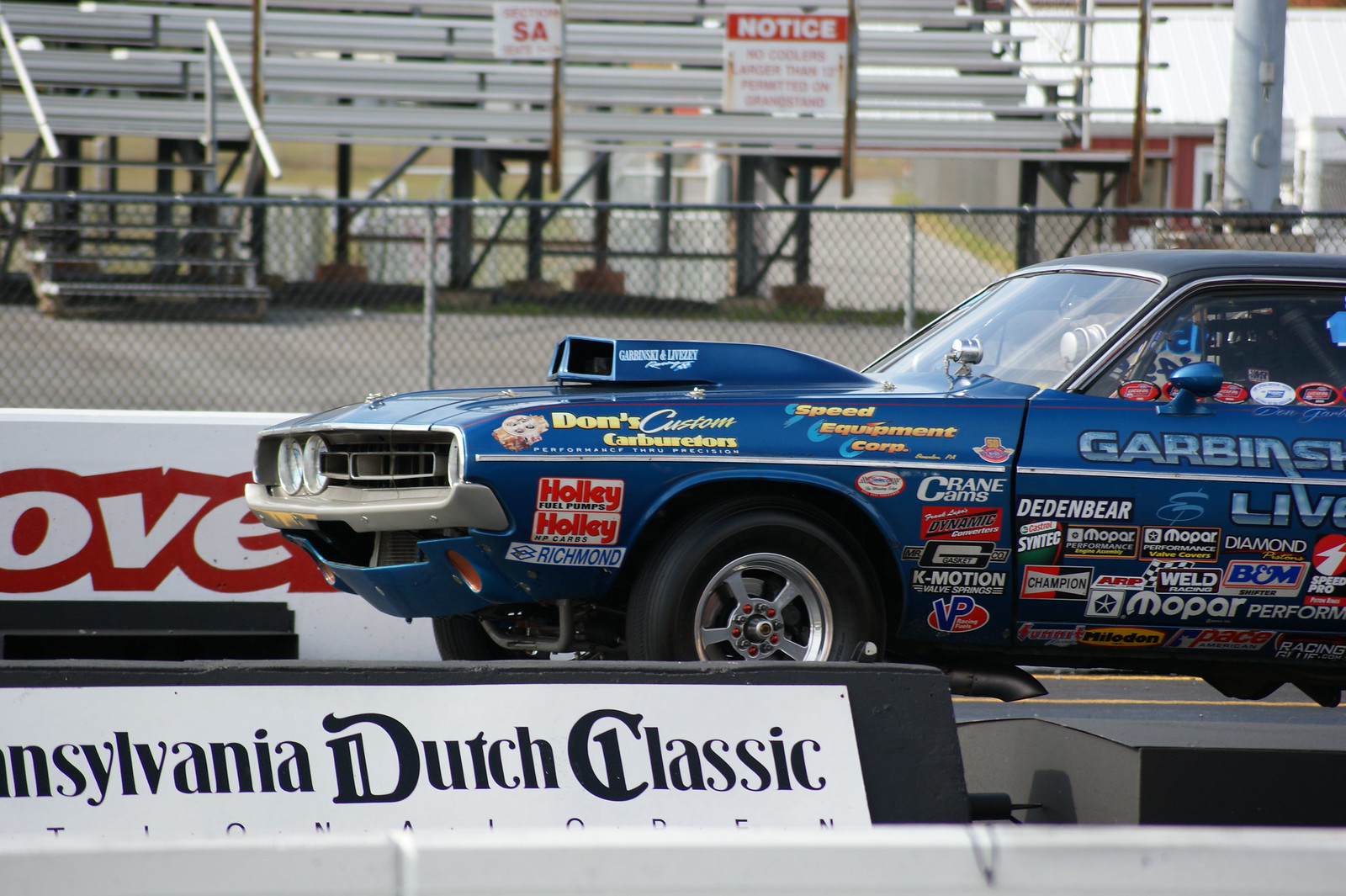This detailed photograph captures a vibrant, royal blue muscle car at a drag racing track, likely from the 1970s. Adorning the car are numerous sponsorship stickers with brands such as Mopar, Crane, K-Motion, and VP, highlighting its race car identity. The image suggests the car is caught in a moment of powerful acceleration, with its front end slightly lifted, indicating the torque lifting it as it takes off. A prominent hood scoop on the driver's side hints at the vehicle's formidable engine. In the background, bleachers and a fence with a notice sign are visible, adding to the race track setting. Adjacent to the car's left is a white barrier with a red graphic, and to the bottom left, a black barrier features a white sign with "Pennsylvania Dutch Classic" in an old-timey font. The scene is illuminated by a sunny day, possibly at an event where the car is on display rather than mid-race.